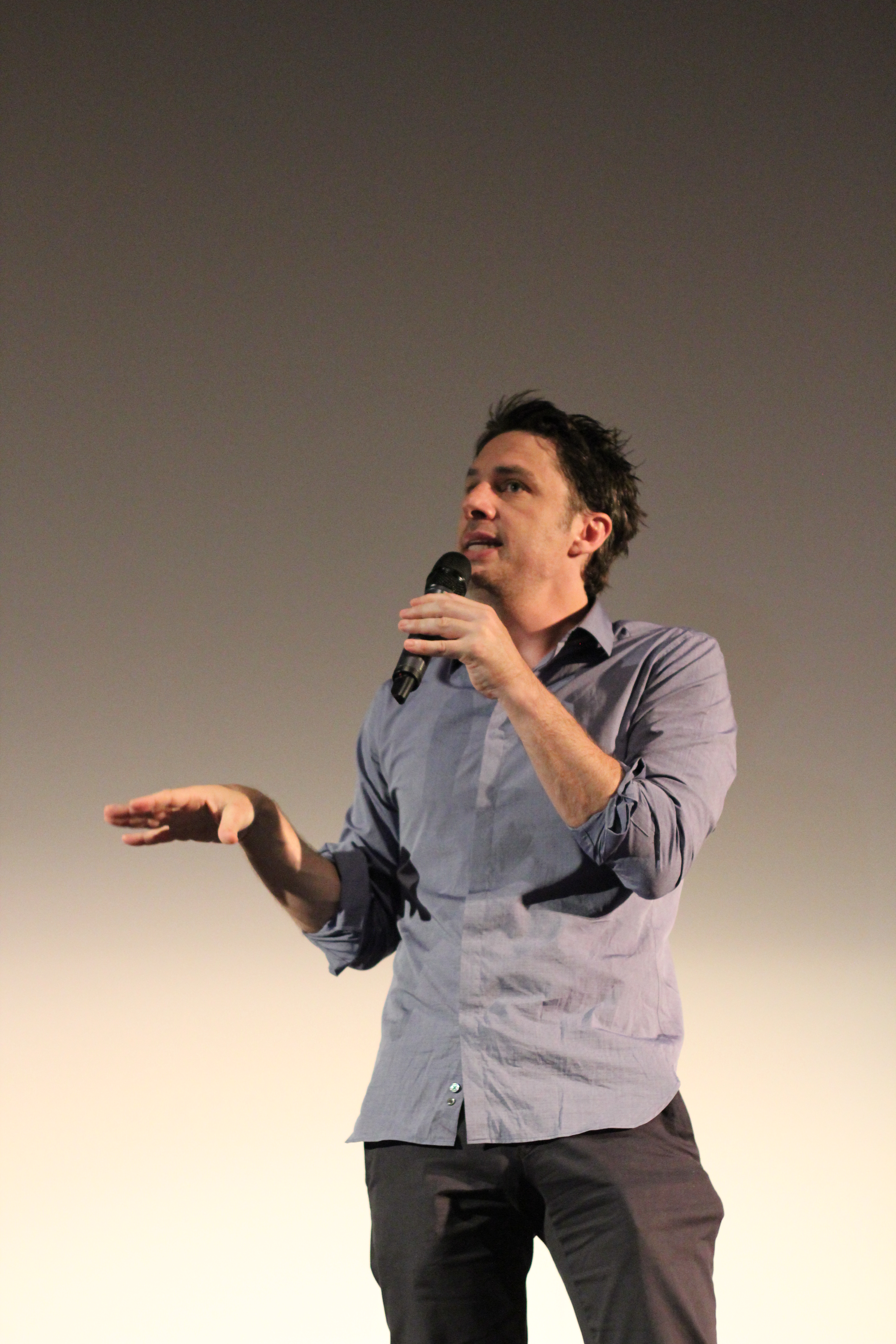This is a detailed photograph of a man who closely resembles actor Zach Braff, standing prominently against a gradient backdrop that transitions from a dark gray at the top to a bright white at the bottom. From the upper calves to the top of his head, the man is dressed in dark gray pants, which noticeably outline several blocky objects in his pockets, likely a wallet or phone. His light gray long-sleeve button-up collared shirt is worn with the top button undone, and the sleeves rolled up to just below his elbows. His short brown hair appears neatly brushed back. In his right hand, he holds a black microphone near his mouth, while his left hand is extended outward, palm down, as he appears to be mid-speech. The background provides no additional context or signage about the location.